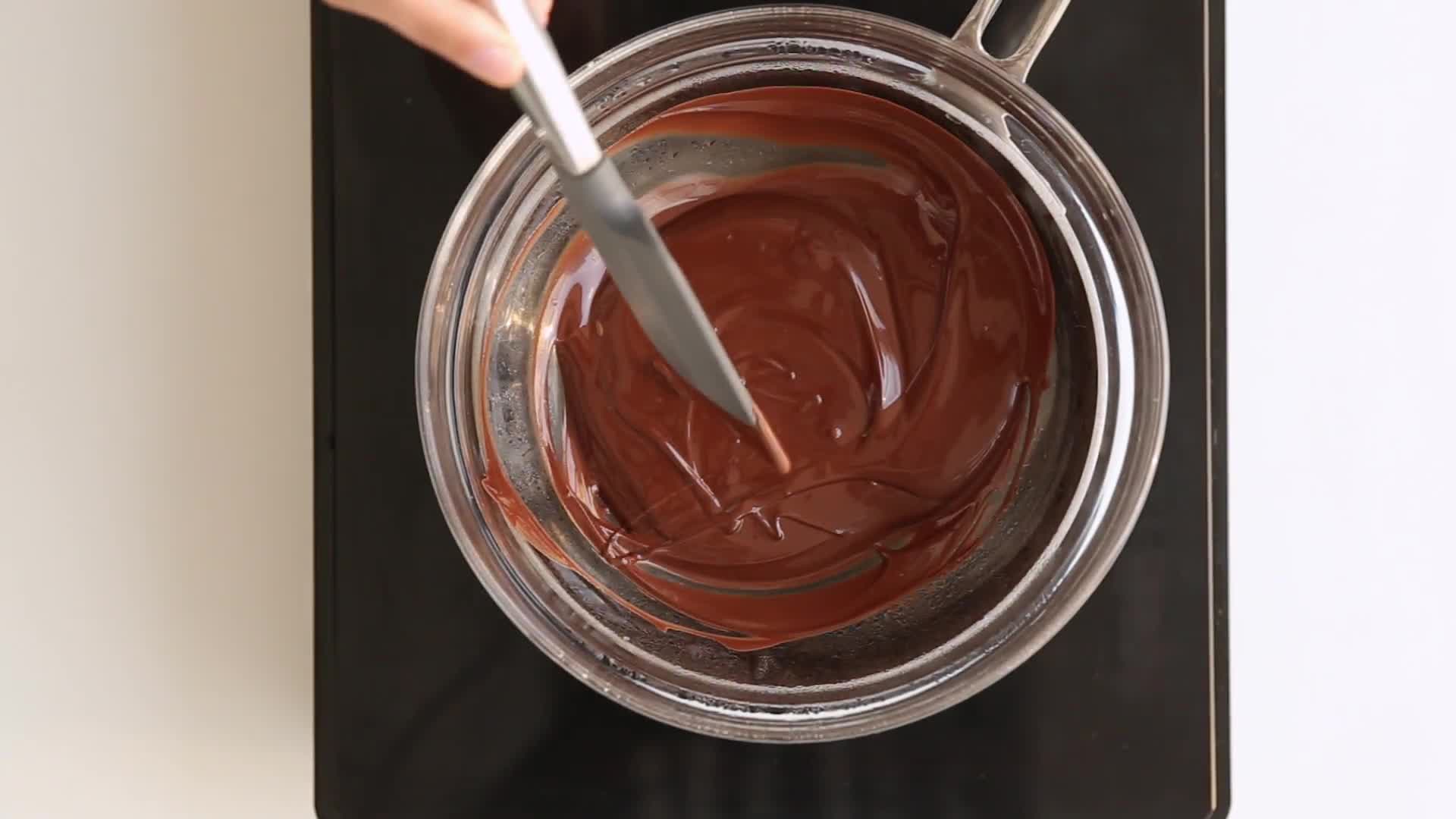In the photograph, we see an overhead view of a double boiler setup on a black electric stove. At the bottom, there's a silver metal pan partially filled with boiling water. Resting on top of the pan is a clear glass bowl containing smooth, melted chocolate. The chocolate appears to be a rich, creamy milk chocolate that is being continuously stirred with a gray rubber spatula to prevent burning. Only the tips of the person's fingers holding the spatula are visible. The image is taken in a landscape orientation, showing the black stove surface and a white border on the right side, with a tan border on the left. The setup indicates that the person is either making a chocolate sauce or pudding using the double boiler method.